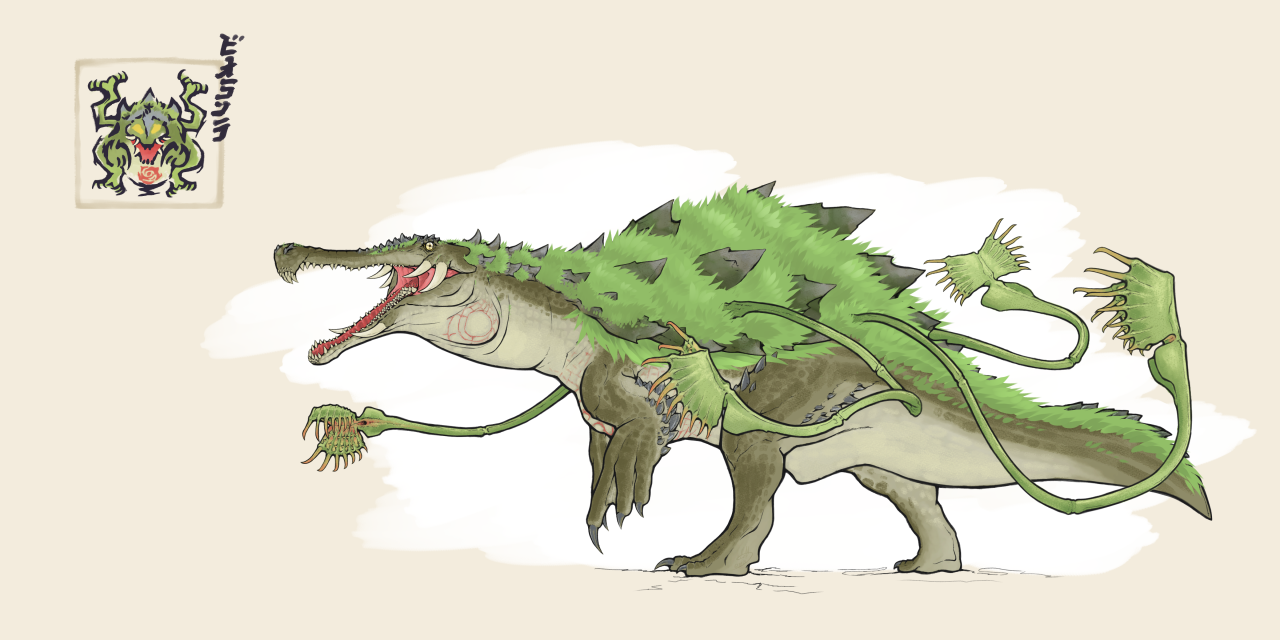The image features a hand-drawn, mutant creature resembling a crocodile, set against a cream-colored background. The creature stands on its two hind legs, with short, flipper-like front limbs. Emerging from its back are four long, vine-like arms that resemble Venus flytraps, with large leaves at their tips. Additionally, the creature’s back is adorned with shark fin-like scales protruding through the grass. The figure is surrounded by a white cloud, accentuating its outline. There’s a logo in the top left corner, accompanied by a small, blurry, vertically-oriented word in black, making it difficult to read. Overall, the scene evokes a fantastical, children's storybook atmosphere.